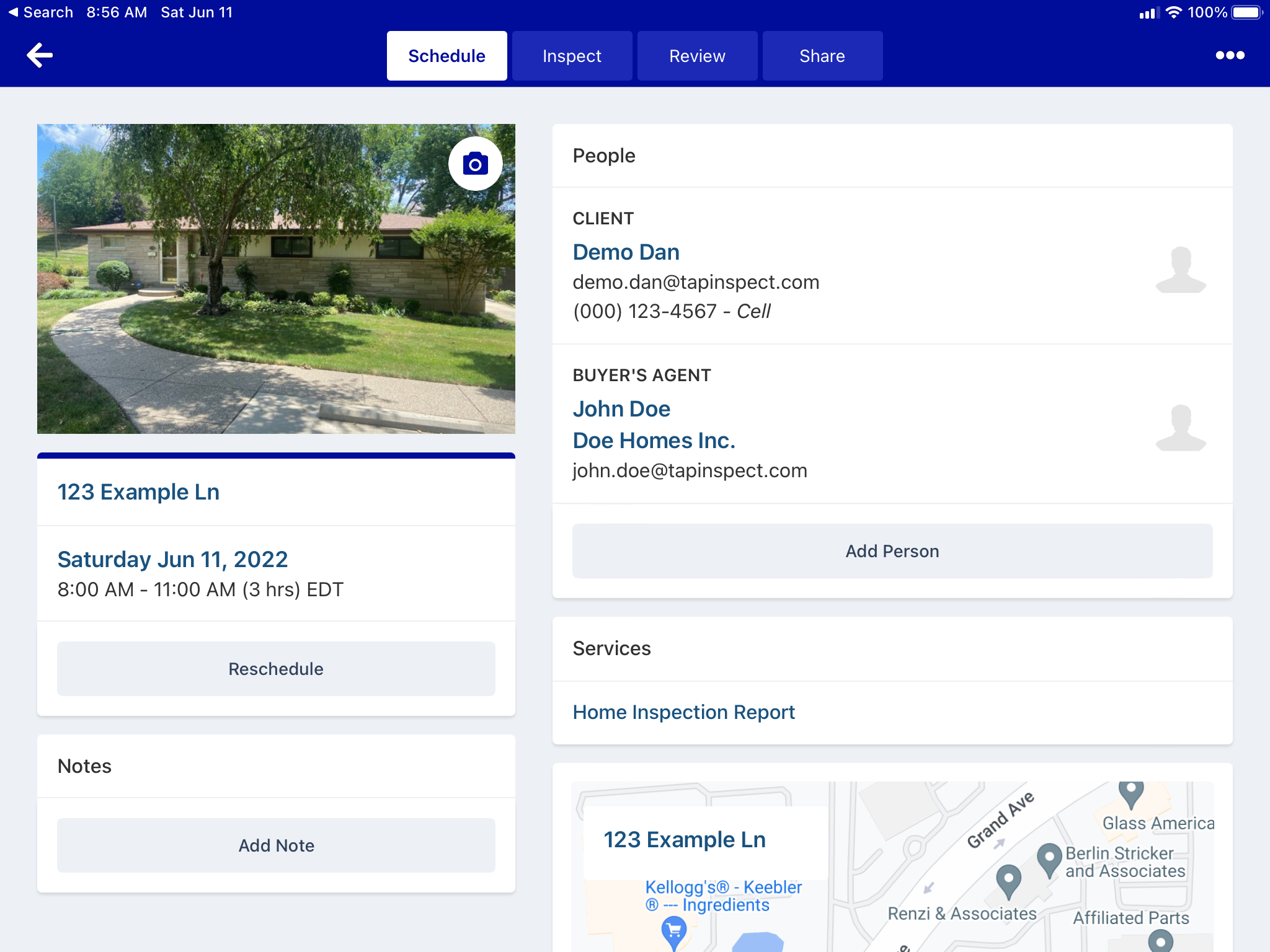**Detailed Caption:**

The image showcases a screenshot captured from an iPad, with notable elements predominantly arranged towards the top left. At the top, the word "Search" is visible in small white text. Adjacent to this on the left is a white play button. Moving to the right, the timestamp "5:56 AM" is displayed, followed by the date "Sat June 11". Below this, a menu bar with a dark blue background features a bold white arrow pointing left on the far left side, indicating a navigation option.

In the center of the menu bar, various menu options are listed, each separated by a space. The selected option, "Scheduled", is marked with blue text and a white background, differing from the others, which have a blue background and white text. The subsequent menu options include "Inspect", "Review", and "Share".

Beneath the menu bar is a section with a light gray background. On the left, there is an image depicting a scenic pathway bordered by a weeping willow tree. Slightly to the right of this image, a flat condo is visible with a bush in front of it and a tree nearby. The condo features approximately three windows and a screen door oriented towards the right.

Further to the right of the image, there is a square area with a white background. At the top left of this section, the word "People" appears in bold gray lettering above a subtle gray divider line. Below this, "Client" is written in bold gray capital letters. The name "Demo Dan" is prominently displayed in bold blue text beneath "Client", with the email address "demo.dan@tapinspect.com" in smaller, non-bold gray text underneath. To the right of the name and email, a gray silhouette of a user represents the placeholder for a profile image. Below this silhouette, the phone number "(000) 123-4567" is listed, followed by another slash and the word "Cell" in italicized lettering.